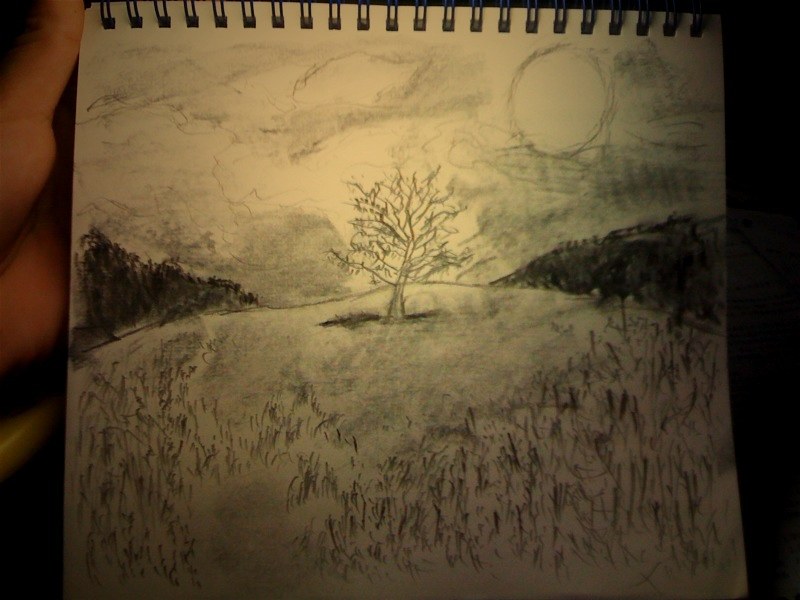The photograph captures a scene with low lighting, featuring a peach-colored cloth fabric as the backdrop. Resting on this fabric is a spiral-bound drawing notebook, oriented so that the rings are positioned at the top of the page. The drawing on the paper appears to have been created using a charcoal pencil. 

The composition of the drawing includes a central hill that spans horizontally across the middle of the page. At the top of this hill stands a solitary tree, characterized by a rounded canopy with numerous branches and sparse leaves. The area beneath the tree is shaded to give depth and dimension. 

The hill itself is sparsely detailed, with just a few lines suggesting the presence of grass. Flanking this central hill are two additional hills, one extending to the left and the other to the right. These hills are shaded much darker, almost to the point of appearing black.

In the sky above the hills, a circle represents the sun. The area immediately above the hills is shaded darker, while the sky transitions to a lighter shade, likely the natural hue of the paper with some subtle cloud forms sketched lightly to complete the scene.